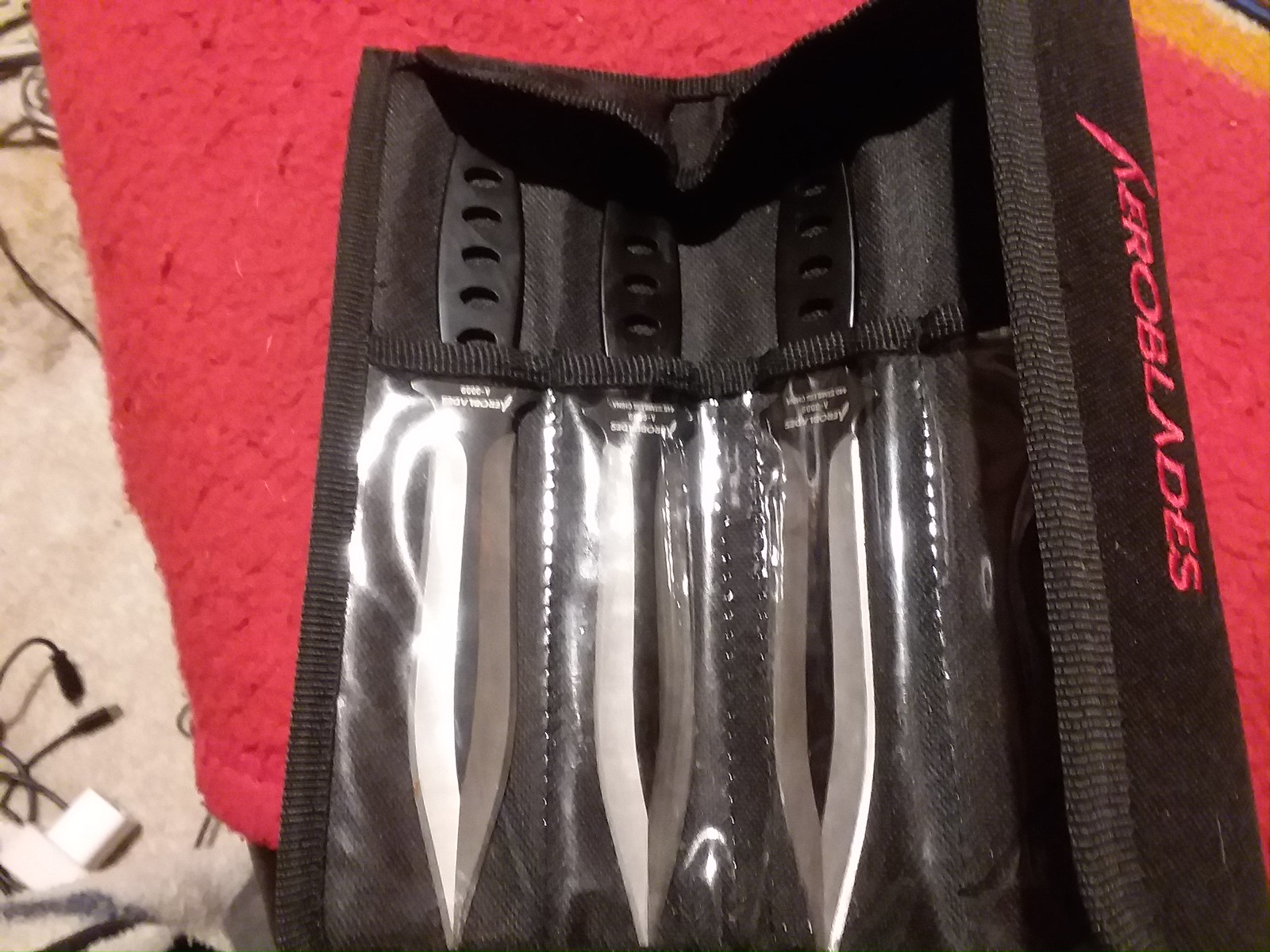In this detailed color photograph, we see an open black nylon case, designed for holding throwing knives, prominently occupying about three-quarters of the image both in height and width. The case features three identical knives, each securely sheathed in clear plastic compartments, revealing their gleaming silver blades and black handles with aerodynamic holes. The case, which can be rolled up and fastened with Velcro, bears a vertical red logo on the right side, reading "caroblades." 

This knife set rests on a multi-layered background: a vibrant red fabric with a yellow stripe at the top edge and a partially visible white fabric with a subtle black floral design underneath. In the lower left corner of the image, there is a small white square object, possibly a cell phone charger. The scene suggests these items are laid out on a bed due to the layers of fabric and intimate setting. The overall composition highlights the sharpness and design of the knives while providing context through its detailed and colorful backdrop.